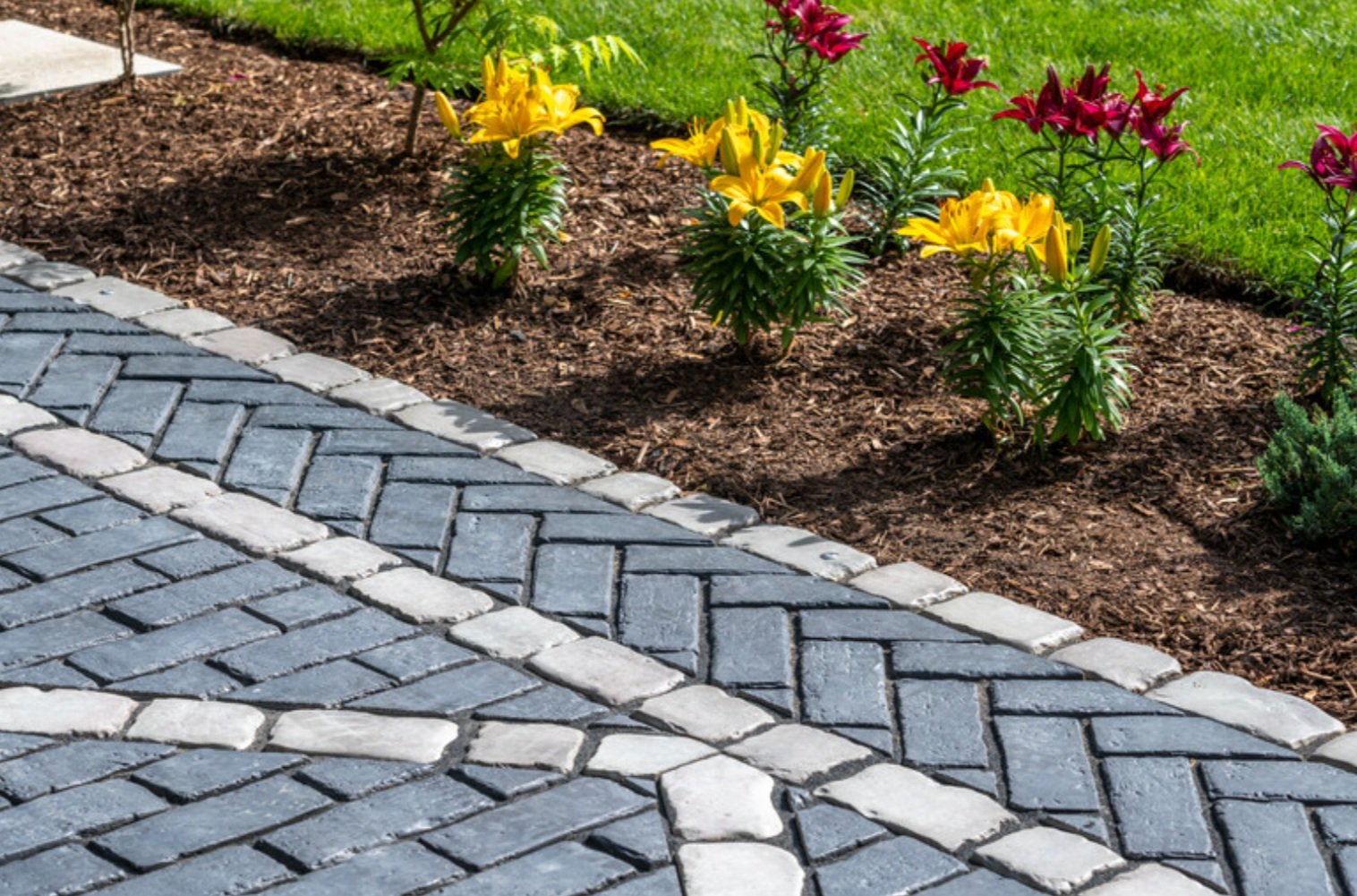This image showcases a detailed view of a walkway or patio constructed with a meticulous brick pattern. In the bottom-left corner, the bricks are primarily a grayish-blue hue, interspersed with white bricks that form a distinctive straight line cutting through the center. These white bricks also appear at a 45-degree angle, creating a triangular pattern that intersects with a perpendicular white line, enhancing the geometric precision of the design.

As the eye moves to the upper right-hand corner, the scene transitions into a vibrant flower bed comprised of brown mulch and soil. This garden area features an array of green plants punctuated by yellow and red flowers, resembling the structure of pineapples with stubby, green leaves leading up to the colorful blooms. The flowers and plants provide a lively contrast to the structured bricks and add organic textures to the scene.

In the top right of the image, a grassy lawn extends upward, providing a lush green backdrop to the structured walkway and colorful flower bed. The upper left corner reveals a small patch of cement, adding to the diverse textures and materials within the image. The sunlight casts gentle shadows across the bricks, highlighting the intricate patterns and natural elements of the garden space. Overall, the scene depicts a harmonious blend of human-made designs and natural beauty, captured in a sunlit outdoor setting.